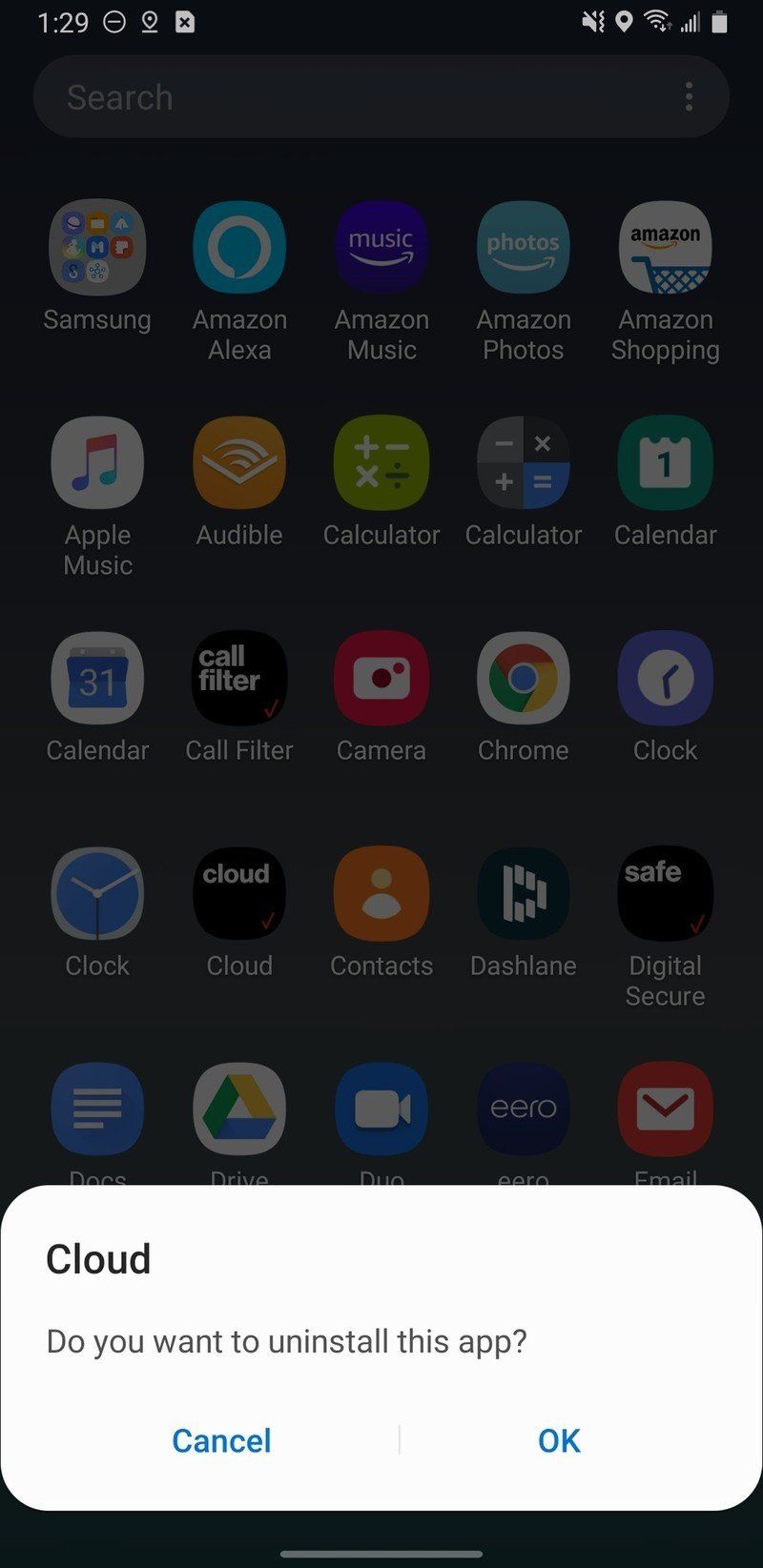The screenshot captures the app drawer of a Samsung Android phone, with numerous applications arranged in a grid layout. Prominently in the foreground is a pop-up window confirming the user's intent to uninstall the app "Cloud", which is symbolized by a square icon with the word "Cloud" inscribed on it. The options "OK" and "Cancel" are presented for user confirmation. The background shows a variety of other apps including Alexa, a collection of Samsung apps, Amazon apps, Apple Music, Audible, Calculator (appearing twice), Calendar (appearing twice), Dashlane, Contacts, Call Filter, Docs, and Clock. The screen also features a search bar at the top for quick navigation through the extensive list of applications. The scene strongly suggests the device is a Samsung smartphone, though the specific model is not identifiable.